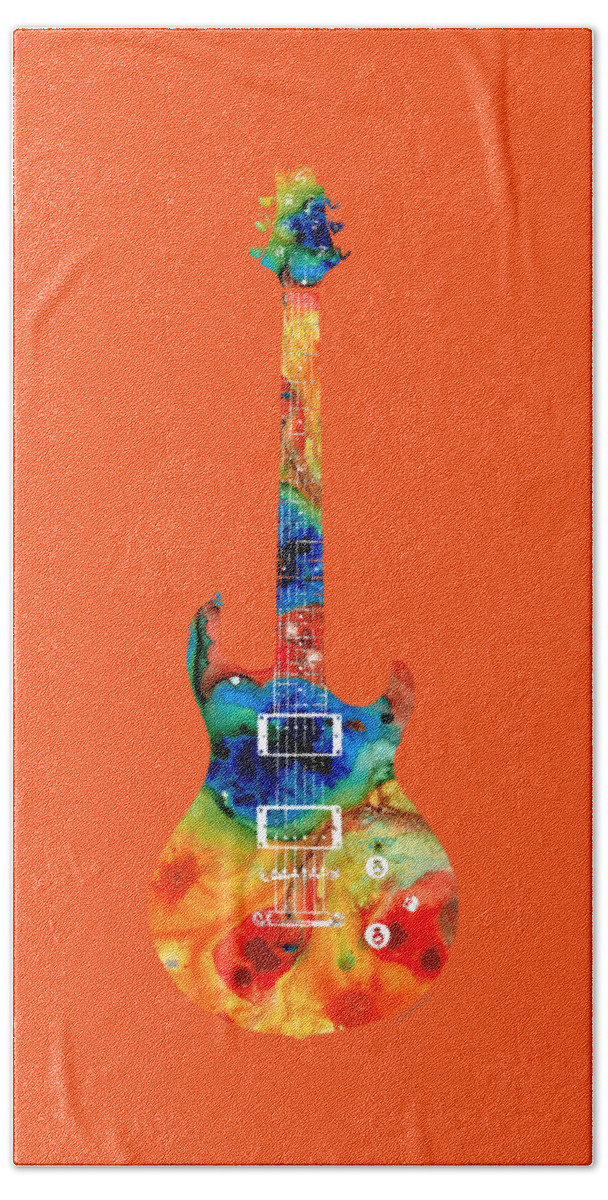This photographic-style image captures a vibrant painting of an electric guitar rendered on what appears to be a rectangular orange fabric canvas, accentuated by noticeable wrinkles. The guitar, positioned upright in portrait mode, boasts a spectacular array of psychedelic, tie-dye colors. Its body features swirling patterns of red, orange, and green, transitioning seamlessly to blues and greens towards the top. The neck of the guitar is adorned with bands of orange and blue, culminating in a head painted in blue and green hues. The strings, frets, and knobs are depicted in white, providing a stark contrast to the vivid color scheme. The painting, devoid of any legible text, beautifully blends traditional guitar shapes with a lively palette that enhances its visual appeal.